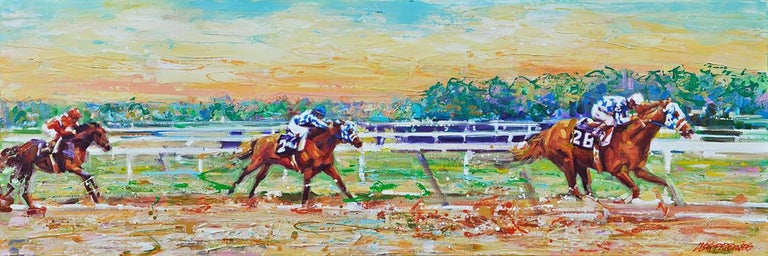This painting depicts a dynamic scene reminiscent of the Kentucky Derby, with three horses galloping at full speed along a racetrack. The horses, painted in earthy brown hues, are spread apart across the canvas: one near the right edge in a jockey's checkered white shirt, one slightly off-center to the left in a blue and white uniform, and the third near the left edge in a red and white outfit. The horse in the lead bears the number 28 on its saddle.

These thoroughbreds are captured in mid-stride, their jockeys leaning forward with intense focus, helmets gleaming in white, blue, and red. The racetrack beneath them is rendered in brownish tones, with flecks of red where the horses' hooves churn the dirt into the air, suggesting palpable motion and speed. A white fence runs parallel to the track, behind which stretches a grassy field dotted with trees.

The distant horizon features a striking sky layered with hues of blue, yellow, and dark orange, suggesting either dawn or dusk, and adding to the painting’s vivid energy. Above the grassy expanse, the sky transitions into varying shades of blue, with hints of white and yellow, suggesting an interplay of sunlight and clouds. In the bottom right corner, the artist's signature can be seen in red.